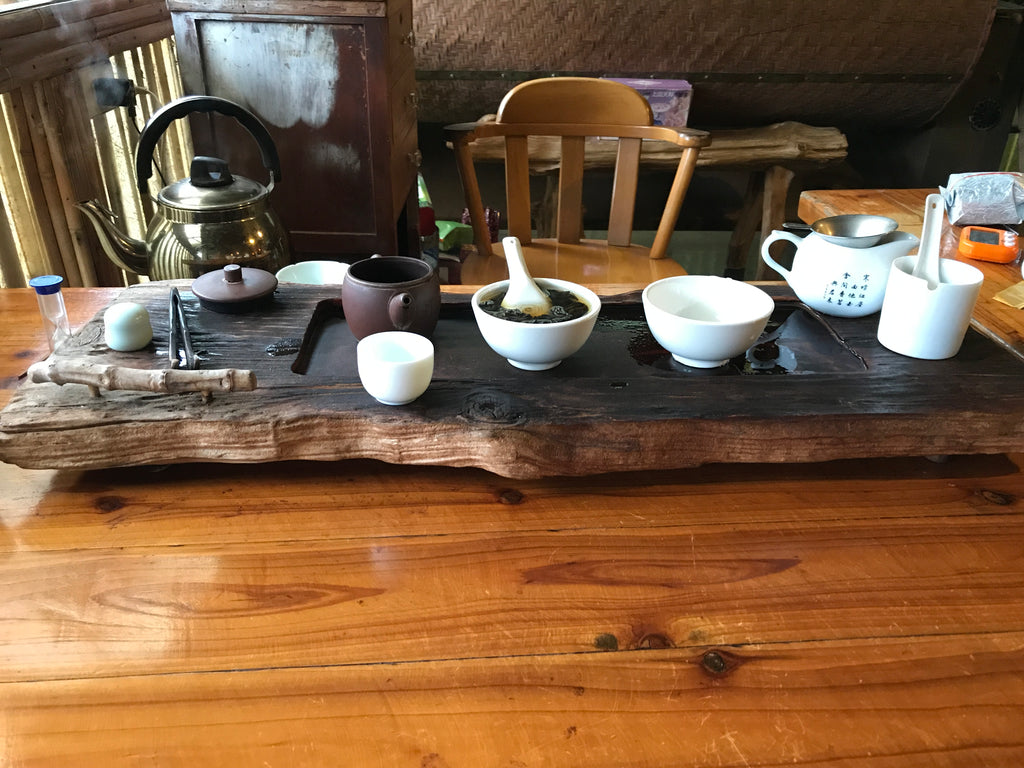The horizontal rectangular image is a richly detailed photograph of a dimly lit room, characterized by an abundance of wooden elements. At the center of the scene is a wooden table with a smaller wooden platform on top. On this platform, a collection of various ceramic objects is meticulously arranged. Dominating the composition are a brown teapot and a white, handleless teacup, along with a white bowl and a mortar and pestle filled with a dark brown substance. A distinct metal funnel protrudes from another teapot. Positioned on the left side of the setup is a glass vial with a blue top, adjacent to the lid of a ceramic pot and what appears to be a stick tool. A chrome teapot with a black handle peeks out from behind the edge of the platform.

The background features a brown, possibly stone wall, accentuated by curtains framing a window on the left. A wooden chair with a slatted back sits behind the table, adding to the room's rustic feel. To the right, another table extends into the background, contributing to the layered and textured scene. An outlet is discretely visible in the upper left corner of the wall. The room's ambiance is created through a muted color palette that includes various shades of brown, black, white, silver, orange, and purple, reinforcing the homely and possibly workshop-like setting.